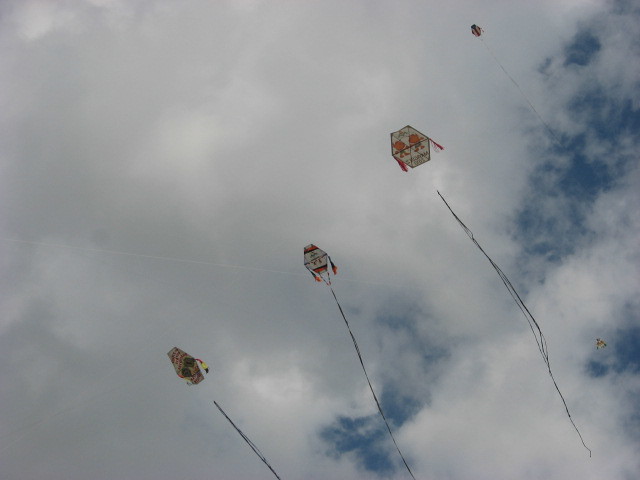This photograph captures a skyward view on a cloudy day, with a predominantly overcast sky punctuated by occasional patches of blue. The clouds are mostly gray and white, creating a moody backdrop. The image prominently features five kites of varying sizes and shapes, encountered while looking up from the ground. The kites are distant but discernible, exhibiting traditional Asian designs with geometric shapes such as hexagons and triangles, primarily decorated in black, white, red, and orange colors. Some kites display intricate ornamentations, including figurines and decorations. Long tails hang from each kite, with one string adorned with black ribbons. A jet contrail spans the sky horizontally in the background, adding an intriguing element to the scene. The overall view suggests a cultural and perhaps festive occasion, where these kites symbolize more than mere children's toys.